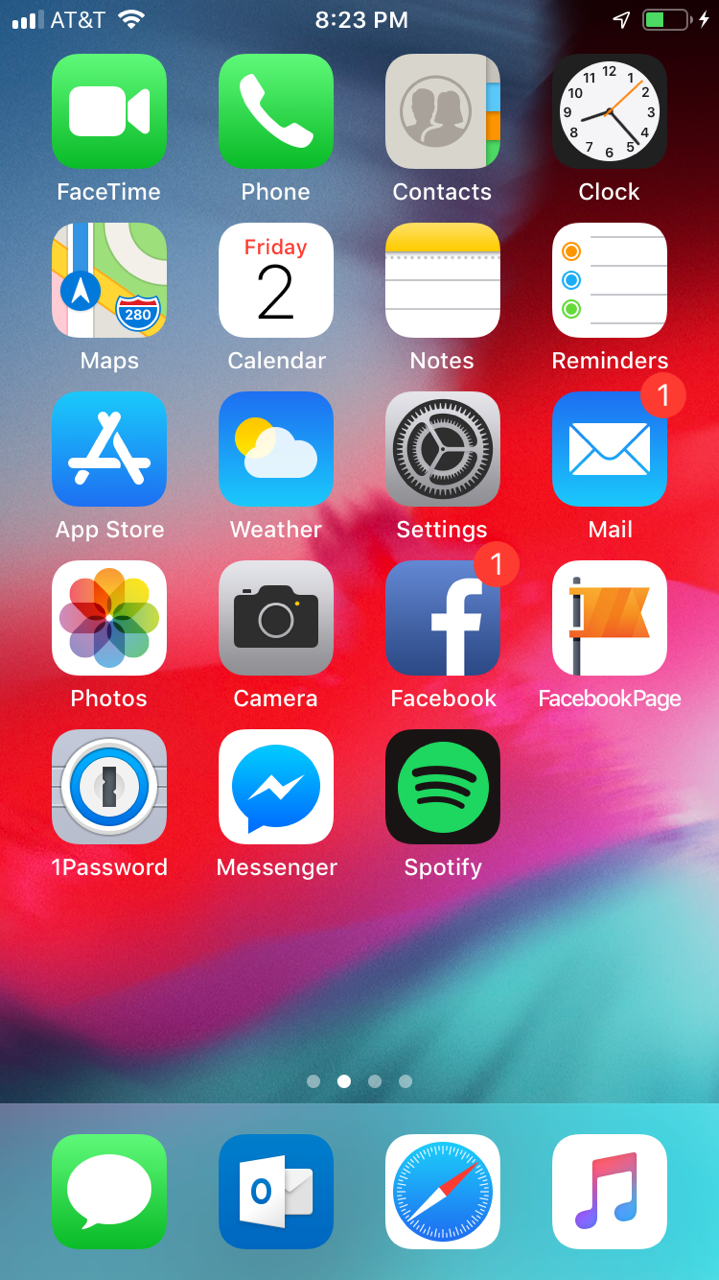The image showcases the secondary home screen of an iPhone, displaying an organized grid of app icons. The visible apps include FaceTime, Phone, Contacts, Clock, Maps, Calendar, Notes, Reminders, App Store, Weather, Settings, Mail, Photos, Camera, Facebook, Facebook Pages, 1Password, Messenger, and Spotify. The screen is indicated to be the second of four total screens, which is noted at the bottom of the display.

The dock at the bottom of the screen houses four main apps: iMessages, an unidentified Microsoft app, Safari, and Apple Music. The background features a vibrant gradient wallpaper blending shades of red, teal, purple, and pink. 

At the top of the screen, the status bar indicates that the phone is connected to AT&T, shows the time as 8:23 PM, notes that the location services are enabled, and displays the battery level at just under 50%, highlighted with a green battery icon.